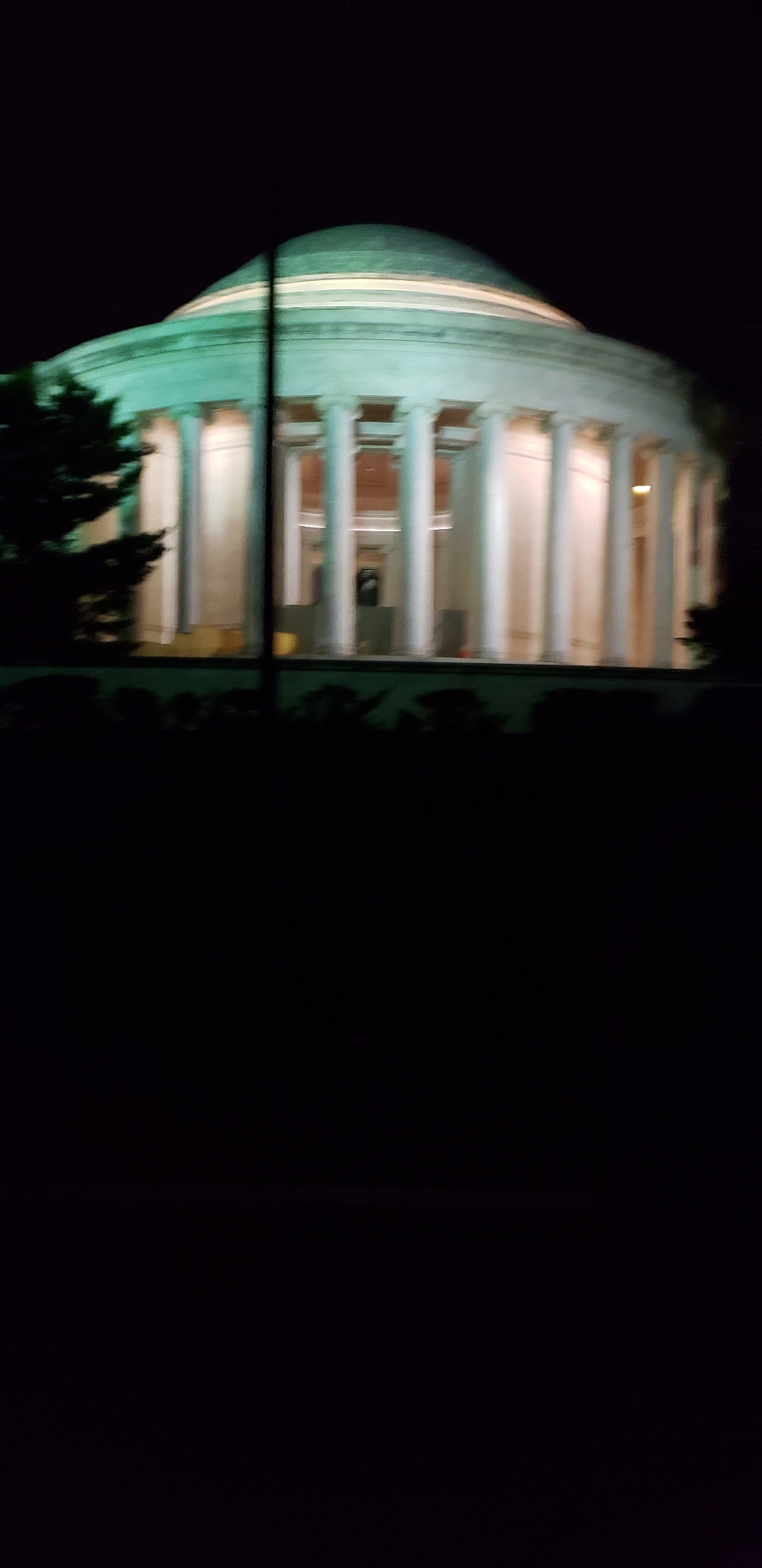This nighttime image captures an outdoor scene dominated by a dark, almost entirely black, background. At the center of the composition stands a stone structure, seemingly ancient and monumental in design. The building features round columns that support a circular stone platform. Atop this platform sits a stone-colored dome, softly illuminated with a yellowish hue around its base. The light from the dome casts a gentle glow on the stone walls mingled with shadow, giving the structure a mysterious, almost ethereal quality. To the left of the structure, the faint silhouette of a tree can be discerned, while a utility pole stands prominently in the foreground, slightly obstructing the view of the structure. The image, steeped in darkness, focuses the viewer's attention on the illuminated building, creating a striking contrast in the nighttime scene.